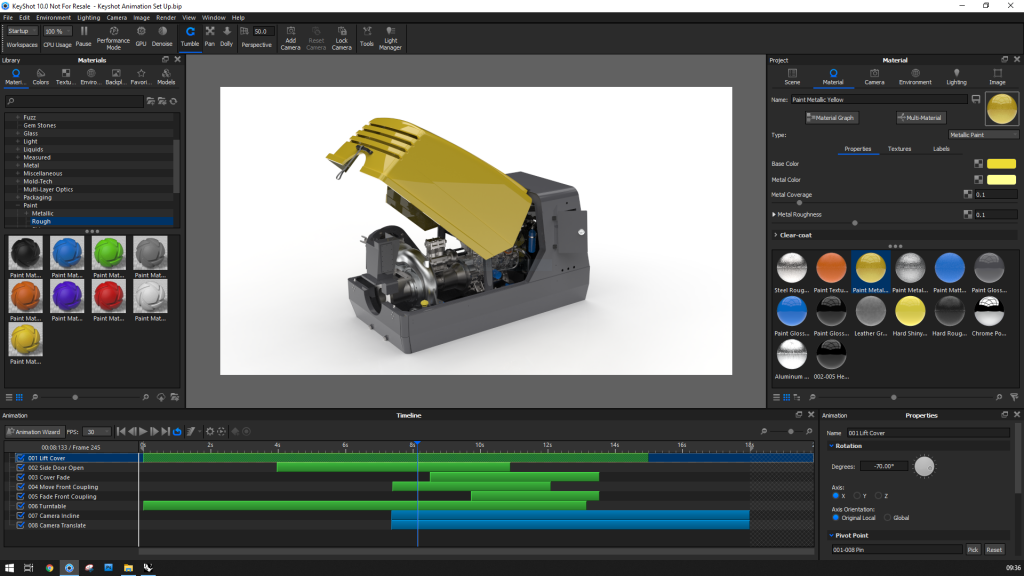This image is a detailed screenshot of a computer-aided design (CAD) program. At the center of the screen is a rectangular metal object, likely an electrical component, featuring a yellow or gold cover and a gray base. Inside the cover, which is open and pointing upward, there are several wires and cords. Surrounding this central image are different sections of the software interface. On both the left and right sides of the screen, there are color palettes with various circular and orb-like images. The top of the screen features multiple menus and possibly a browser or control panel in the top left corner. The bottom of the screen displays a series of green and blue bars, which resemble graphs or activity indicators, potentially representing project timelines or other data visualizations.